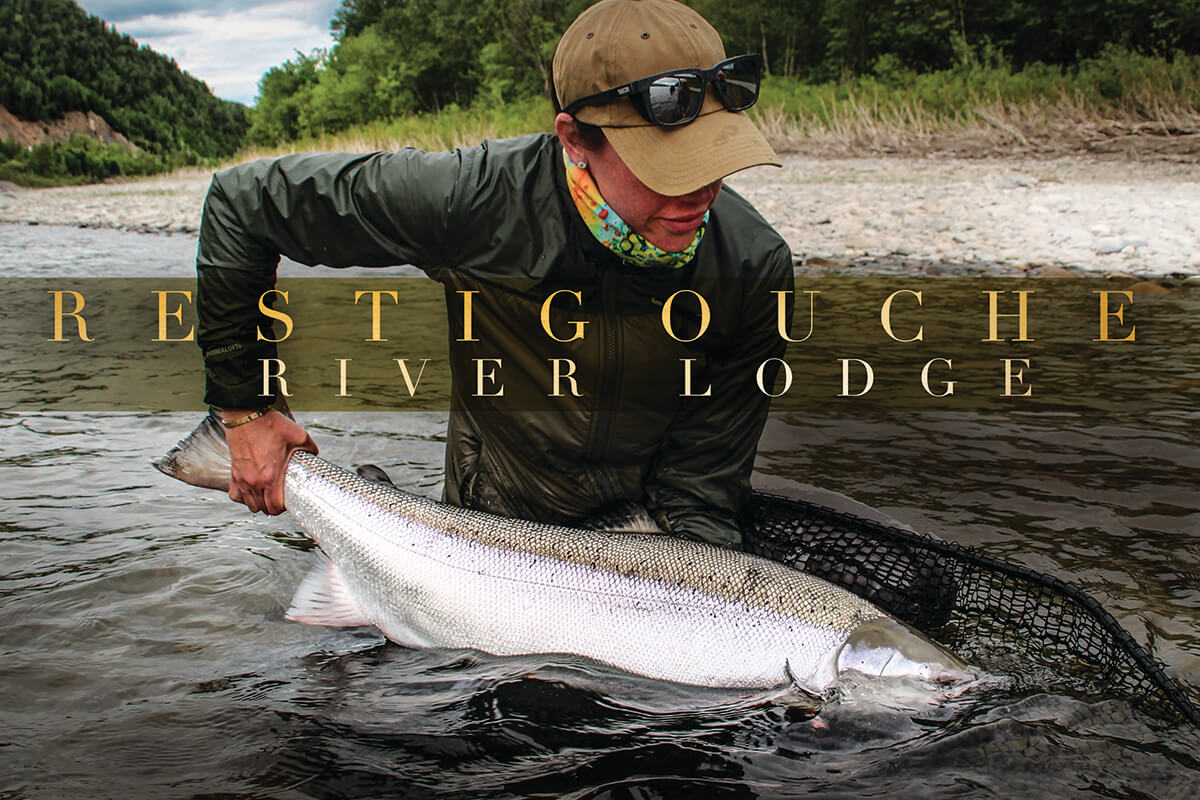The image is an advertisement for Restigouche River Lodge. Prominently featured in the center are the golden capital letters spelling out "RESTIGOUCHE" with "River Lodge" in white text beneath it. Positioned behind the text is a woman in a river, wearing a brown baseball cap with sunglasses resting on top and stud earrings. She is clad in a dark suit with a scarf around her neck. The woman is holding a very large fish horizontally with her right hand gripping its tail, while the fish’s head is partially submerged in the dark green water. A black net, likely used to catch the fish, is visible on the right side. The backdrop consists of leafy greenery, sandy pebbles, and rocky areas near the shore. Further back, the scene includes dried brush, green grass, and a mix of trees and hills, with patches of blue sky and scattered clouds peeking through the vegetation.